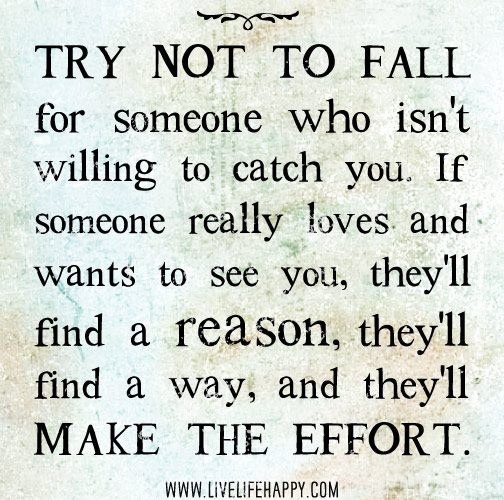This is an inspiration graphic sourced from www.livelifehappy.com. The background features an antiqued paper texture rendered in a mixture of light green, blue, and sepia tones, giving it an aged, mottled appearance. Adorning the very top center is a delicate filigree design. The central message, displayed in black font, reads: "Try not to fall for someone who isn't willing to catch you. If someone really loves and wants to see you, they'll find a reason, they'll find a way, and they'll make the effort." The initial phrase "Try not to fall" and the concluding phrase "make the effort" are emphasized with larger capital letters. Below the main text, centered at the bottom, is the website's name in black: www.livelifehappy.com.